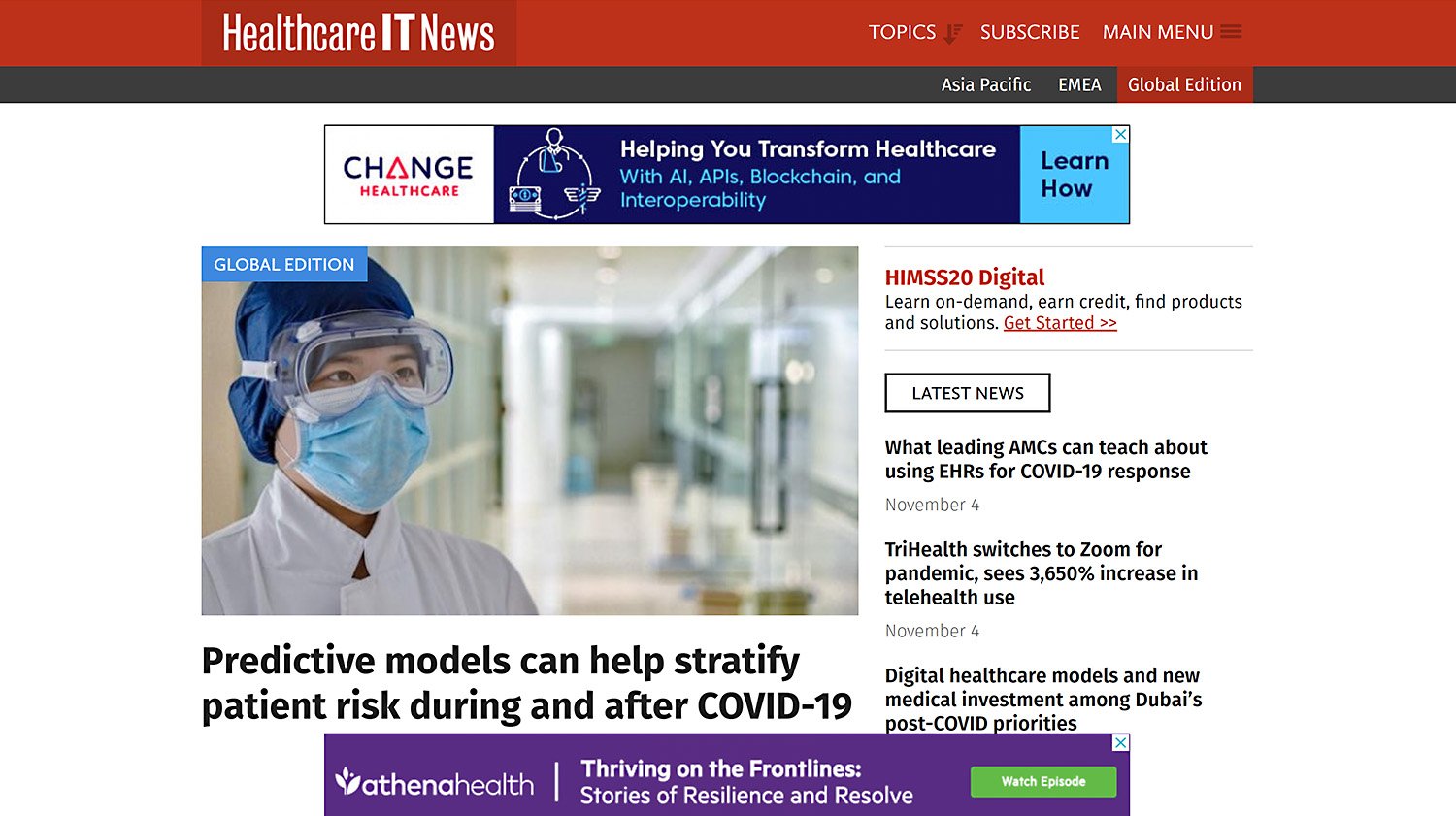**Detailed Caption for Healthcare Website Banner Image**

The image showcases a banner perfectly suited for a healthcare or news website. Dominating the top section is a dark red rectangle featuring an inset maroon red rectangle, slightly offset to the left. Within the maroon red section, white text reads "Healthcare," followed by "IT" in bold white, and concludes with "News" in standard white font.

To the right, there are various navigation tabs: "Topics," symbolized by a maroon red thermometer icon, "Subscribe," and "Main Menu," which is represented by three black lines indicating expandable options. Beneath this, there's a dark black bezel containing white text labels: "Asia Pacific," "EMEA," and a red rectangle marked with "Global Edition."

Further below, on the left, a white section labeled "Change" features a distinctive red triangle for the letter A, while the "CH" and "NGE" are in blue text. Directly underneath, in red text, it reads "Healthcare." Adjacent to this, in dark blue, a message reads "Helping You Transform Healthcare," followed by cyan-blue text "With AI, APIs, Blockchain, and Interoperability," with each letter of "Interoperability" spaced out for emphasis.

At the rectangle's end, a cyan-blue portion contains a gray box with a blue "X," and the text "Learn More" in black. Below this banner, an image portrays a lab assistant in a hospital setting, wearing a dark blue scrunchie, cyan-blue mask, white lab coat, and blue-rimmed safety goggles. Black text at the bottom states, "Predictive Models Can Help Stratify Patient Risk During and After COVID-19," while red text to the right reads "HIMSS20 Digital." Underneath, in black text, it says, "Learn On-Demand, Earn Credits, Find Products, and Solutions," followed by an italicized red "Get Started" with two rightward arrows underlined.

Next, a rectangular section with a black border reads "Latest News." Black text enumerates: "What Leading IMCs Can Teach About Using EHRS for COVID-19 Response" dated "November 4th" in gray, "TriHealth Switches to Zoom for Pandemic, sees 3,650% increase in telehealth use," also "November 4th in gray," and "Digital Healthcare Models and New Medical Investment Among Dubai's Post-COVID Priorities."

A purple rectangle follows, displaying a leftward leaf image and "ATHENA" in bold white letters, next to "Health" and a bold white line. In bold white text, it proclaims, "Thriving on the Front Lines," and regular white text continues, "Stories of the Resilience and Resolve." On the right, a green rectangle with bold white text reads, "Watch Episode." A gray square at the top right exhibits a cyan-blue "X."

This meticulously designed banner effectively combines essential navigation, informative content, and striking visual elements to engage viewers on a healthcare-centric platform.